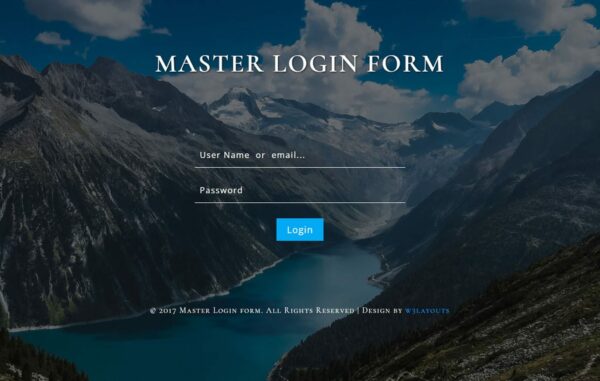The image depicts a screenshot from a website, likely intended for administrative use, displayed in a landscape orientation without any borders. The background is a stunning photograph featuring a dramatic landscape of snow-capped, glacial mountains that steeply descend into a serene, blue lake nestled in the valley below. The slopes of the mountains in the foreground are lush with vegetation, while the peaks in the background are blanketed in pristine snow. Above the mountains, the sky is a vibrant blue, adorned with puffy, white clouds.

Overlaying this picturesque scene, the title "MASTER LOGIN FORM" is prominently displayed at the top center of the image in all capital letters, using a serif font resembling Times New Roman. Below the title, there are a few lines of the unobstructed background photo, followed by a thin white line labeled "Username or Email..." where users are expected to input their credentials. Another thin white line beneath it is labeled "Password," and below this field is a solid blue rectangular button that reads "Log In."

At the bottom of the page, the footer notes "Copyright 2017 MASTER LOGIN FORM. All rights reserved," followed by "Design by [unreadable text in blue]." The textual elements are all rendered in white, except for the designer’s name, which is in blue.